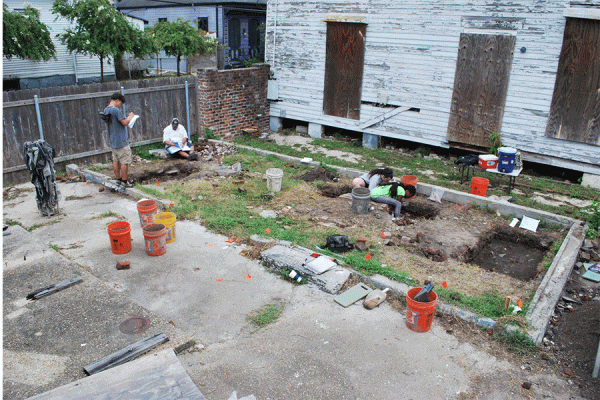The image is a color photograph of a construction site that resembles a backyard area adjacent to an old, wooden house in an urban or suburban environment. The house, painted white with wooden doors, appears disheveled and possibly abandoned, as some doorways seem boarded up. The scene is bustling with activity as four people are working on the site. Numerous orange and yellow buckets, as well as a white bucket, are scattered around, filled with various materials, suggesting significant digging and construction work. In the left part of the image, under a tree branch, a man in a gray shirt and shorts stands, focusing on a book or paper, likely overseeing the project. A second man, dressed in white, sits in front of him on the paved section of the yard, which contrasts with the grassy patches to the right. Two girls sit at the center, examining something on the ground. Noteworthy details include concrete slabs and a blue cooler, implying the workers are prepared for a long day, with their notebooks indicating careful recording of their activities.